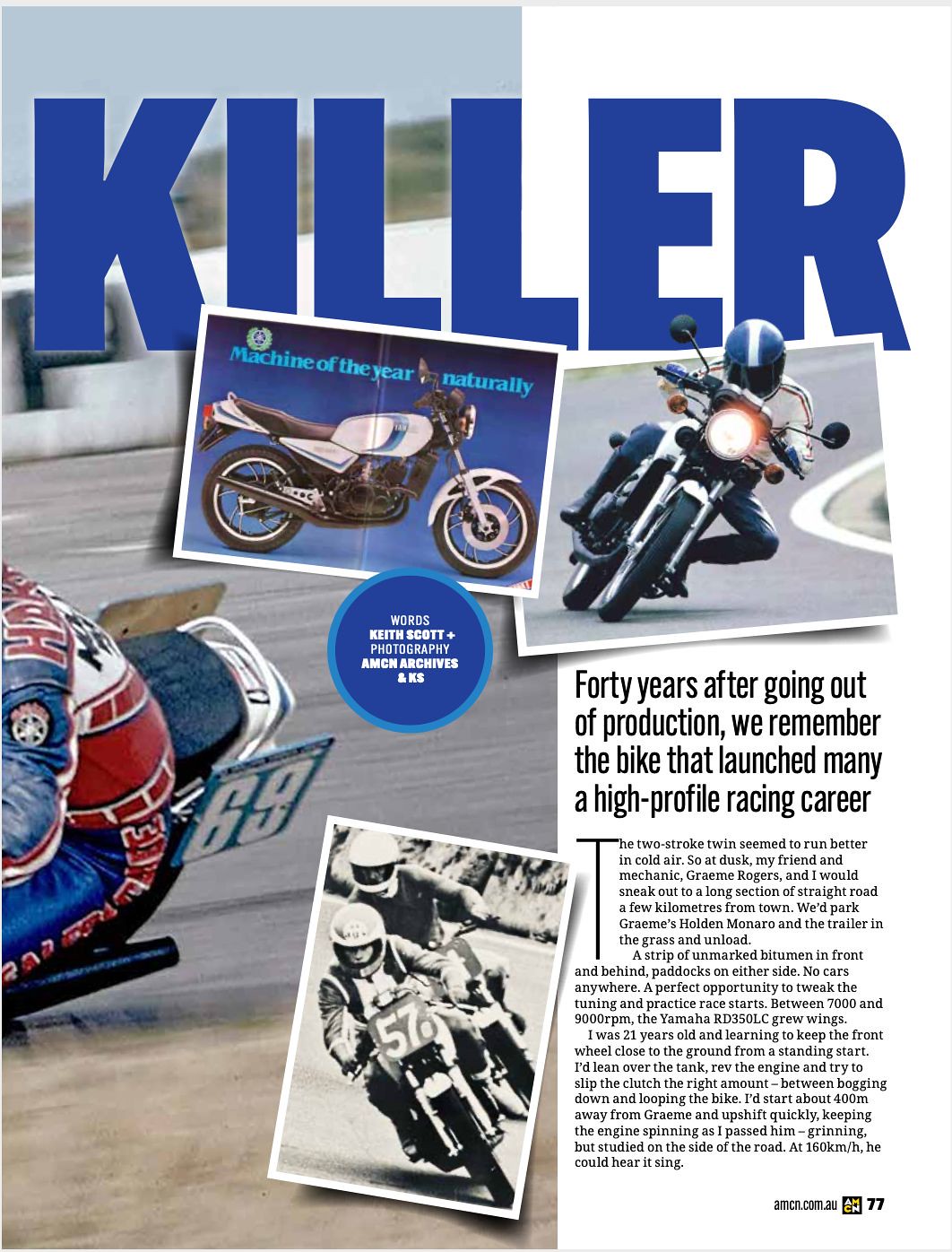This image captures the first page of a detailed motorcycle magazine article titled "Killer," prominently displayed in blue text at the top center of the page. The central focus is on several images of motorcycles and their riders, set against an asphalt backdrop with one rider actively racing. The page features an evocative mix of color and black-and-white photos, including a nostalgic black-and-white image at the bottom. The emphasis of the article is on a legendary bike, celebrating its legacy 40 years after its production ceased. The story recounts the experiences of a young rider mastering the Yamaha RD350LC, highlighting the exhilarating practices held on a deserted stretch of road. The text describes the bike's remarkable performance between 7,000 and 9,000 RPM and the rider's techniques to maintain control at high speeds. This content is positioned on page 77 of the magazine "AMCN," with the logo and URL (amcn.com.au) neatly placed at the bottom right corner.